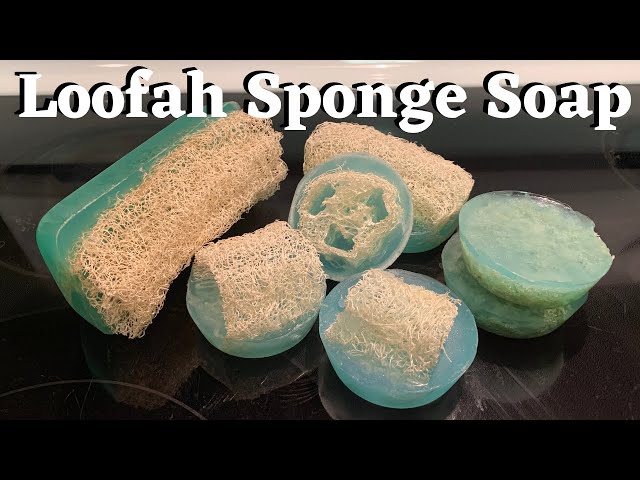The photograph showcases various pieces of loofah sponge soap, arranged on a dark reflective surface. The image features a black background with white text at the top labeling it as "loofah sponge soap." The soaps are green or bluish-green in color, semi-opaque, and translucent, giving them a gem-like quality. There are seven pieces of soap: five are circular, and two are rectangular, resembling traditional soap bars. Embedded in the soap are sections of loofah, a tan, fibrous material, with some pieces of loofah sticking out while others are fully encased within the soap. The loofah provides a textured appearance, with colors ranging from light brown to mossy green, ensuring the soap serves both for cleaning and exfoliating.